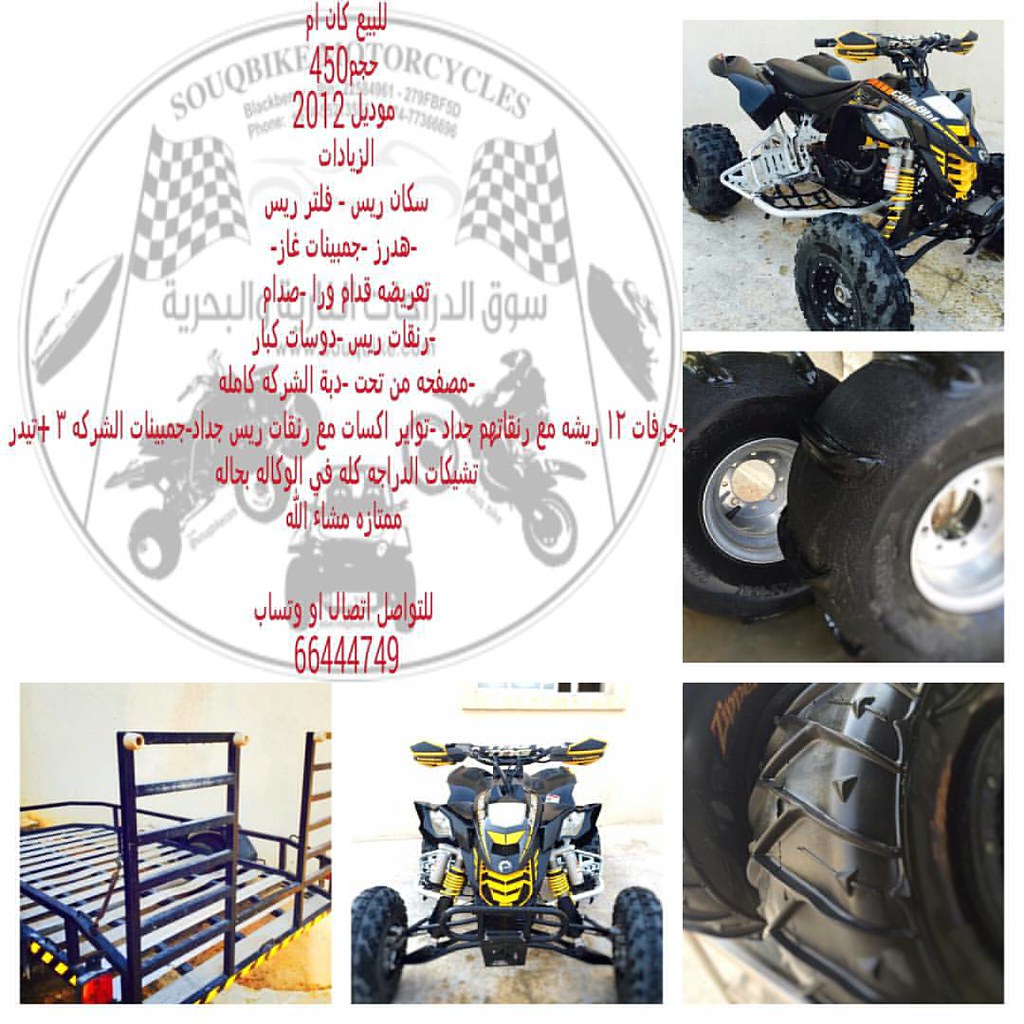The image features a central section with text in a language that appears to be Arabic, framed by five photographs arranged on the left and right. At the center top, there is red text superimposed over what seems to be a circular logo for a motorcycle business, depicting race flags, motorcycles, and ATVs. The photos on the right side include: at the bottom, a close-up of a tire of an off-road vehicle; above it, multiple tires and wheels; and at the top right, a front view of a four-wheel off-road vehicle. On the left side, there is an image of a blue metal motorcycle trailer at the bottom and another off-road vehicle in the bottom center. The imagery suggests a focus on off-road vehicles and motorcycles, emphasizing their components and associated equipment.